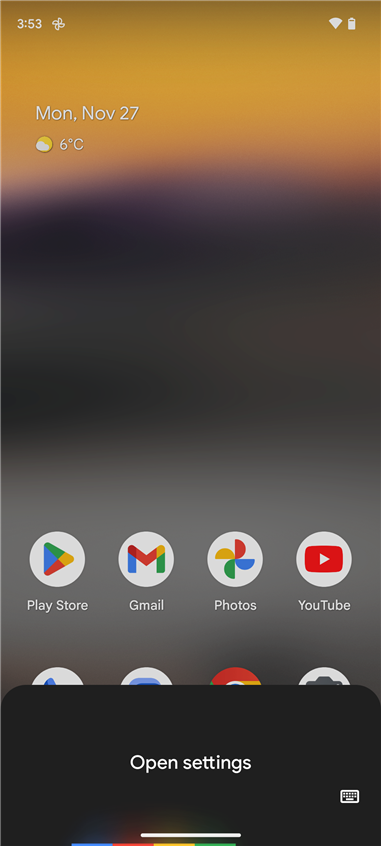The image depicts a thin smartphone, likely a Google device, displaying a screensaver featuring a picturesque sunset. It's Monday, November 27th, and the clock reads 3:53 PM. The Wi-Fi signal is strong, and the battery is fully charged. The temperature is a brisk 6 degrees Celsius, with its details showcased vividly against the brighter sections of the sunset image. The darker part of the sunset fades towards the middle of the screen, which remains clear of any information.

At the bottom of the screen, several application icons are visible, indicating active functionality. These include the Google Play Store, Gmail, Google Photos, and YouTube, with additional icons for a camera app, Google Chrome, and two partially visible icons. Approximately the lower 20% of the screen is occupied by an open settings interface with a small keypad icon, suggesting a prompt to input further commands or settings adjustments.